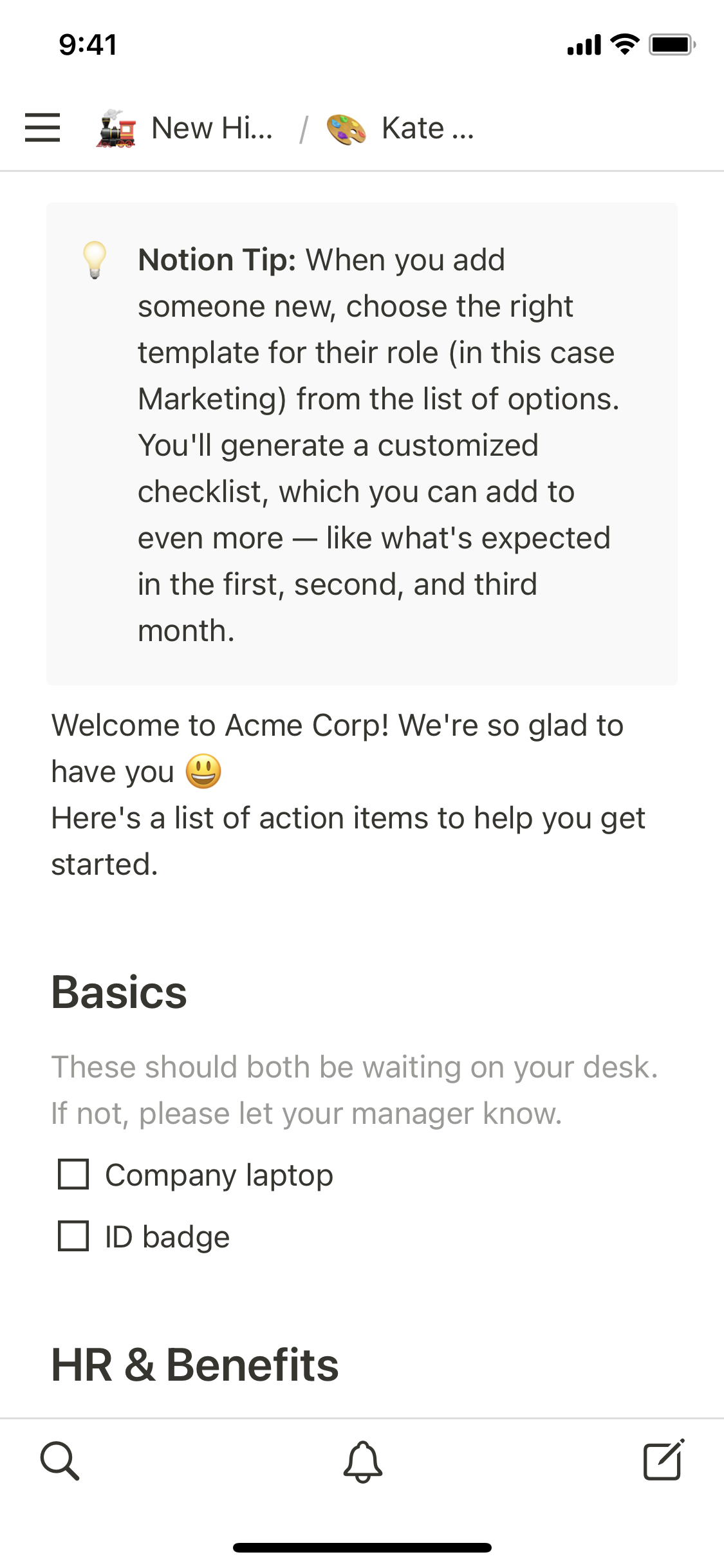A mobile screenshot with a white background and no border, displaying an interface that seems to be part of an onboarding program for a company, likely titled "New Hire." At the top left, the time reads 9:41, while the upper right corner shows two Wi-Fi icons and a fully charged battery. Below this, in the header, there are three horizontal gray lines symbolizing a menu, followed by "New High" (likely "New Hire"), a train icon, a slash, and "Kate."

Below the header, a section with a light bulb icon is labeled "Notion Tip." The main text reads, "Welcome to Acme Corp. We're so glad to have you. Here's a list of action items to help you get started." Below it is a section titled "Basics" in large font, followed by a light gray note: "These should both be waiting on your desk. If not, please let your manager know." Listed are two items with checkboxes: "Company Laptop" and "ID Badge."

At the bottom left, there's a label "HR and Benefits." The footer bar, set against a white backdrop, contains three outlined black icons: a search icon, an alerts icon, and a message icon. A centered horizontal black line runs at the bottom of the image.